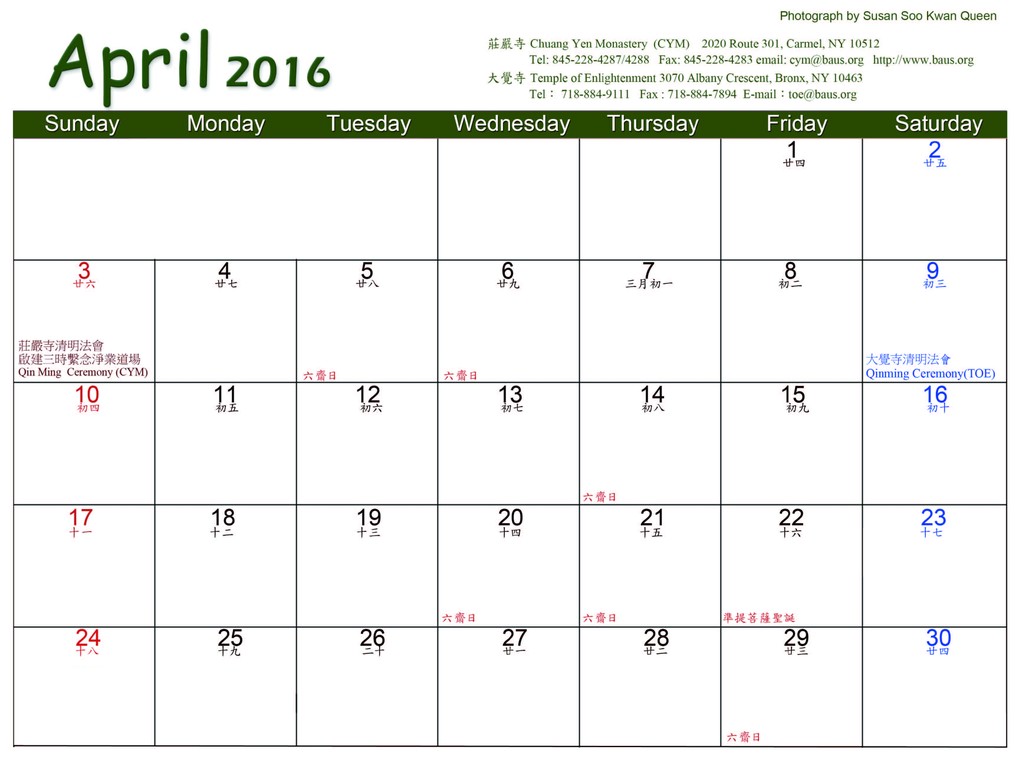This image of a calendar prominently displays April 2016. The days of the week - Sunday, Monday, Tuesday, Wednesday, Thursday, Friday, and Saturday - are shown at the top in white lettering against a dark green bar. The dates for Sunday are in red while the dates for Saturday are in blue; the other days are in standard black. At the top left corner, "April 2016" is highlighted in green.

The calendar is adorned with a variety of details. At the top right corner, it reads "Photographed by Susan Sue Kwan Queen," indicating the photographer. Below this text, there are multiple sections featuring contact information in English and presumably Chinese characters. One section lists "Chinyoung Monastery, 2020 Route 301, Carmel, New York" along with telephone and fax numbers, and an email address. Another section provides similar contact details for "Temple of Enlightenment, 3070 Albany Crescent, Bronx, New York."

The calendar layout includes typical numbered boxes representing the 30 days of April. Notably, some of the days feature additional characters, likely in Chinese, which indicate specific ceremonies occurring on the 3rd and 9th of the month. This diverse textual presentation renders the calendar both functional and richly informative.